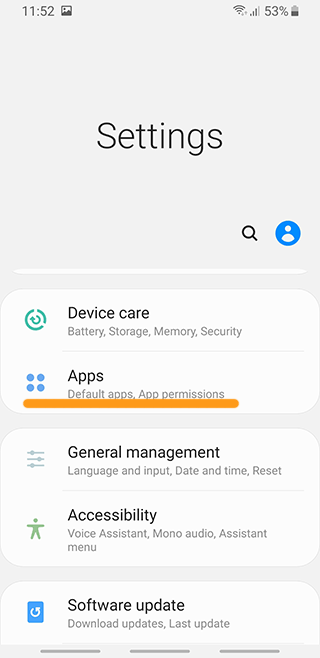The image showcases a cell phone screenshot with a portrait orientation and a solid light gray background. At the top left corner, the time is displayed as "11:52," while the top right corner features standard cell phone icons, including signal strength indicators and a battery icon showing 53% charge.

Centered at the very top of the screen is the word "Settings," accompanied by a small search icon and a profile icon. Below this header, a thin white line spans the width of the screen, demarcating different sections of the settings menu.

The first section consists of a white box with rounded corners, containing two main entries written in black font. The first entry includes a green circle icon labeled "Device Care," which encompasses battery, storage, memory, and security settings. The second entry is titled "Apps" and covers default apps and app permissions, represented by four small blue dots. A thick orange line with rounded corners is situated beneath these entries.

After a slim gray space, the next white box with rounded corners is visible, labeled "General Management and Accessibility." Following this, at the bottom of the screen, a third white box with rounded corners appears, although only its top portion is visible. This section displays "Software Update," along with options to download updates and details regarding the last update.